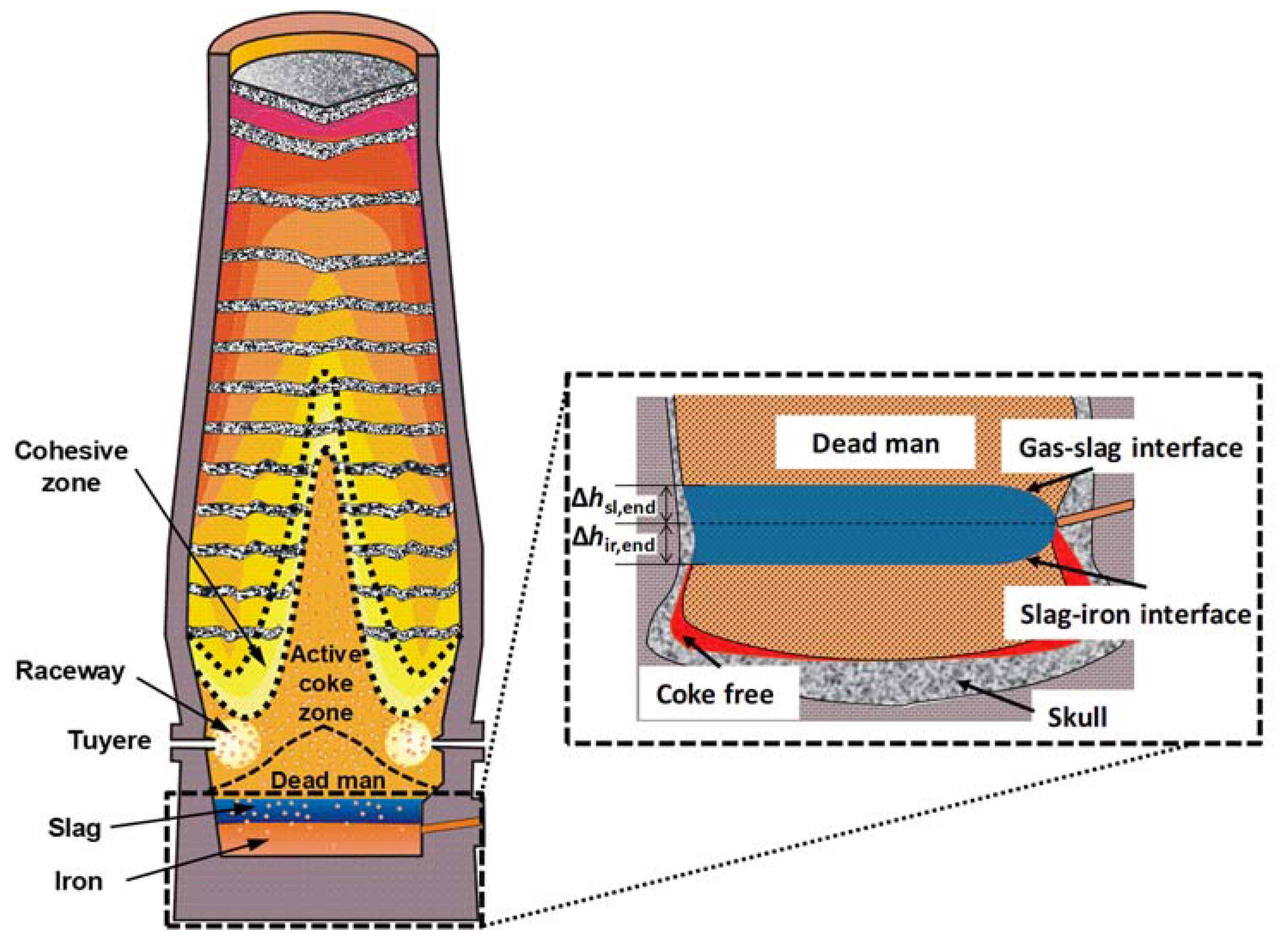The image is an infographic detailing the internal structure and function of a conical iron forge. On the left, a cross-sectional diagram highlights various colored layers within the forge, each separated by gray and black dotted lines. The layers, colored in shades of orange, yellow, and pink, are labeled with terms such as "cohesive zone," "raceway," "two-year," "slag," "iron," "active coke zone," and "dead man." The diagram provides a comprehensive view of the layered and intricate design of the forge. 

To the right, a zoomed-in segment focuses on the bottom part of the forge, marked by critical zones and interfaces. Labels identify the "dead man," the "gas slag interface," the "slag iron interface," and the "skull." A section called "coke free" is highlighted in red, suggesting a specific area devoid of coke. This detailed inset provides an in-depth look at the lower segments of the forge, which are essential in the melting and refining processes.

Overall, the infographic employs a detailed color scheme and labeling system to convey the functional complexities of an iron forge, from the cohesive zone at the top to the "dead man" and slag interfaces at the bottom.